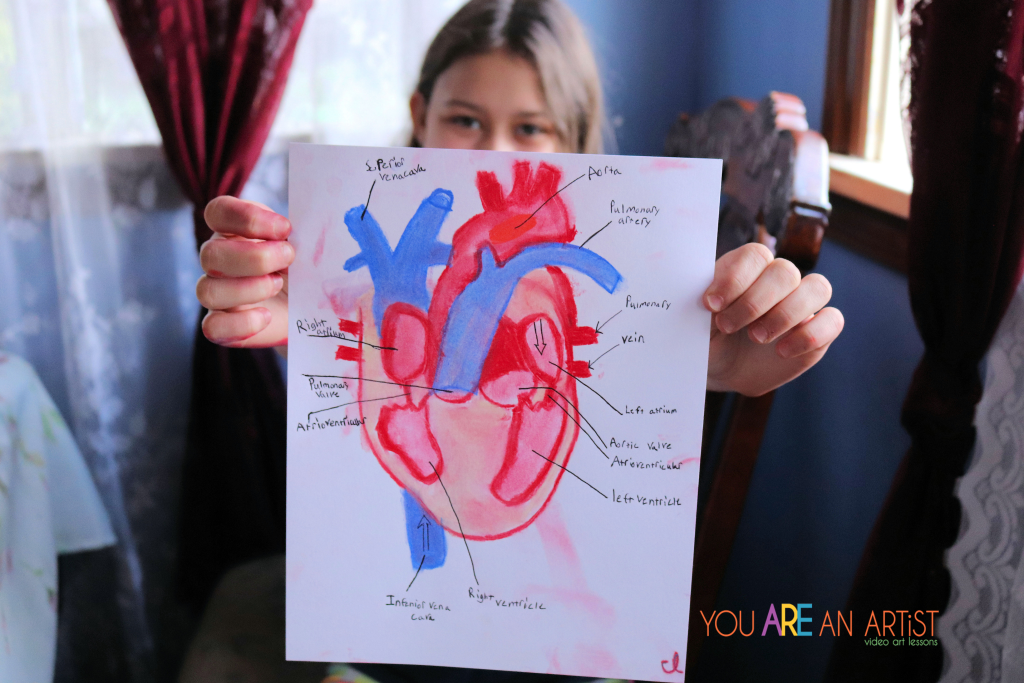The image depicts a young girl, possibly an elementary-aged child, with brown hair and dark eyes, sitting in a wooden chair in a room. She is holding a white piece of paper in front of her face, obscuring everything except her eyes and forehead. The paper features a hand-painted anatomical heart in hues of red, pink, and blue, with black lines and labels pointing to different parts, such as the aorta, pulmonary artery, and ventricles. The background of the room includes dark red curtains and blue walls, with a window visible to the right. In the bottom right corner of the image, the text "YOU ARE ARTIST" is prominently displayed in varying colors: "YOU" in orange, "A" in purple, "R" in yellow, "E" in blue, and "ARTIST" in orange. Below this, it reads "Radio Art Lessons." The overall scene gives the impression of a young artist proudly showing her work, perhaps part of a school or art lesson setting.